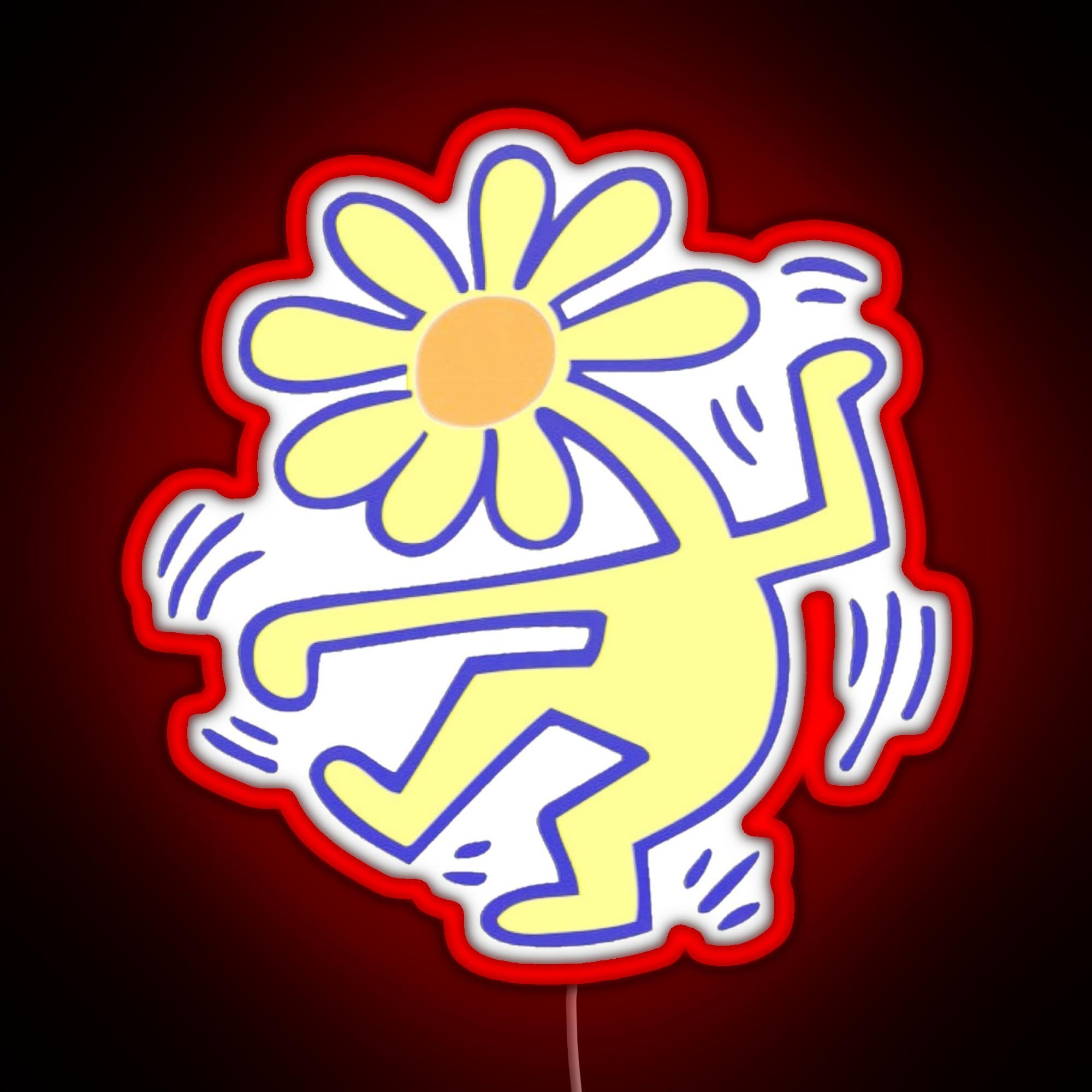This image features a vibrant neon sign set against a burgundy background, which deepens into a dark, blackish-red hue towards the corners. The central focus is a dynamic illustration outlined in red neon tubing, showcasing a cartoon figure in mid-dance. This figure is distinguished by its unique head—a daisy-like flower with orange at its core. The character's body is yellow, presenting a lively dance pose with arms outstretched and bent legs. The interior of the red outline holds a white backdrop, with additional purplish-blue lines depicting the figure's form and energetic movement, accentuated by animated lines indicating motion.